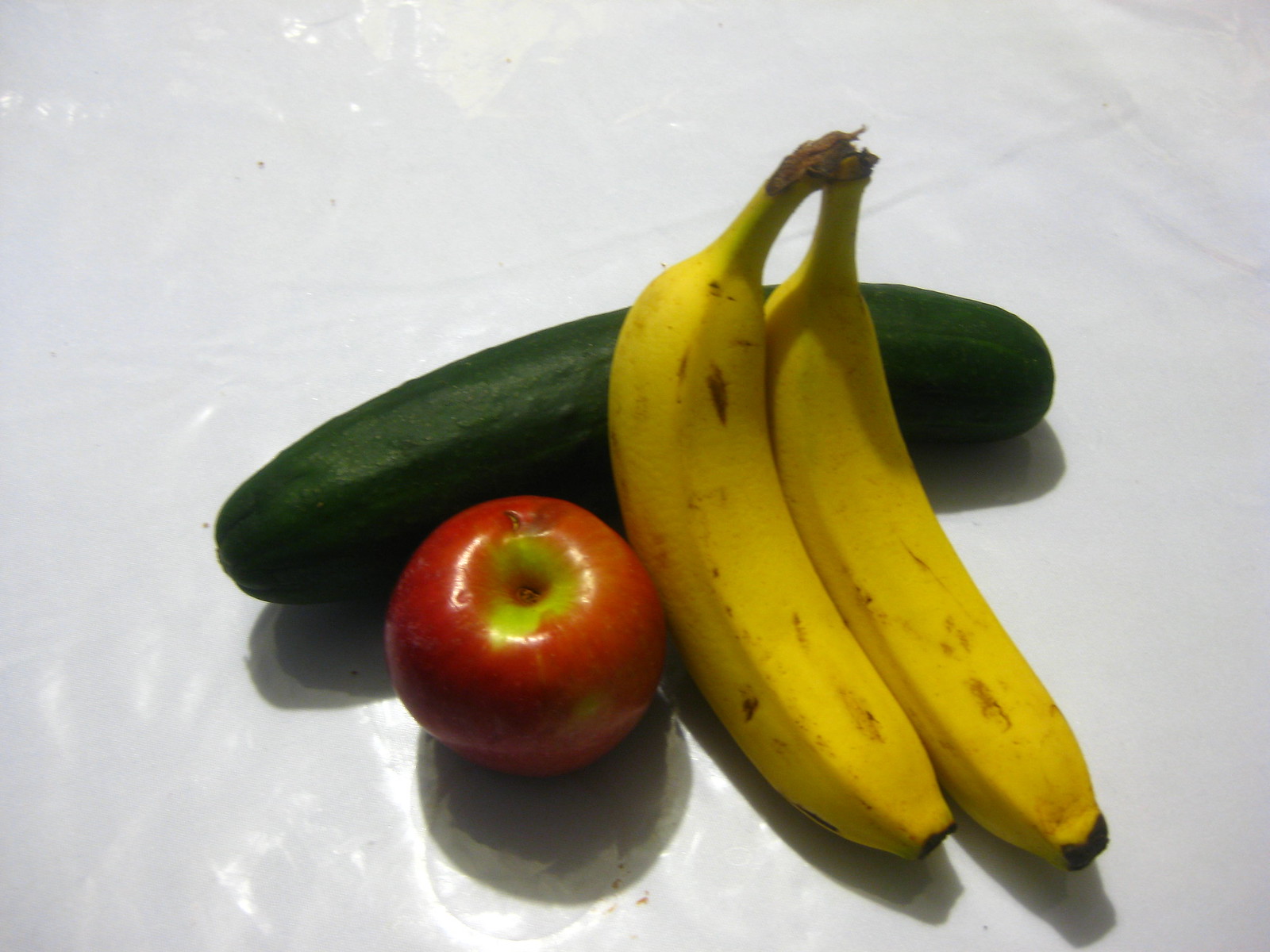A crisp, white surface resembling a paper or vinyl tablecloth, slightly creased and textured, is the setting for a small fruit arrangement. At the center lies a horizontal, dark green cucumber, subtly angled towards the bottom left of the image. Near the cucumber's middle, two ripe bananas rest, their bright yellow skins adorned with a few brown spots and a hint of green near the still-connected stems. The bananas are positioned diagonally, pointing towards the bottom right. To the left of the bananas, nestled in the corner formed with the cucumber, sits a mostly red apple. The apple is missing its stem, revealing a small green spot where it once was. Shadows from the cucumber and apple gently fall on the tablecloth, adding depth to the simplistic composition.